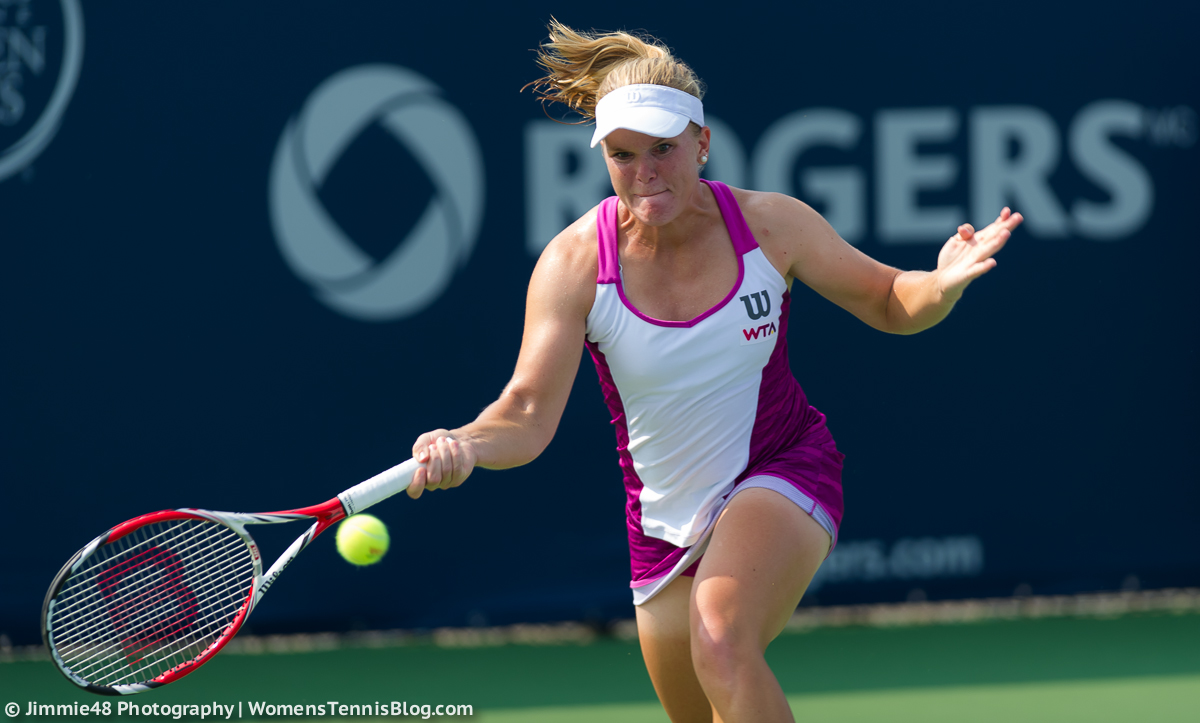The image showcases a female tennis player on an outdoor court during a sunny day. She is positioned centrally, poised to hit an approaching tennis ball. The athlete, a fair-skinned woman with blonde hair pulled back into a ponytail, is intensely focused on the ball with her lips pursed, giving her a determined and almost stern expression. She wears a white visor and a white tennis dress adorned with purple stitching along the sides and top. Her attire includes purple shorts, visible underneath the dress, and a Wilson logo on the front left side of her jersey. 

In her right hand, she grips a red and white Wilson tennis racket, preparing for a forehand stroke, while her left arm extends upwards. The tennis ball is captured in mid-air, directly in front of her racket. The background features a blue advertisement banner for Rogers, with a distinctive circular logo. Additionally, there is a visible copyright notice from Jimmy48 Photography at the bottom left, reading "womentennisblog.com." Below her feet, the court displays a greenish turf, highlighted by the shadows cast by the sun, enhancing the vivid outdoor atmosphere of the scene.